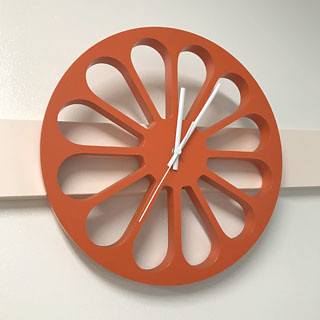The image showcases a modern terracotta-colored clock mounted on a white wall. The clock features an abstract design with 12 petal-shaped cutouts in place of traditional numbers, giving it a floral appearance. The clock hands are white, and the time displayed is 12:05, with the second hand at the 35-second mark. Light filters through the petal cutouts, casting intricate shadows on the wall behind. The clock itself is fixed to a slightly protruding white support board, adding a layer of depth to the setup. The overall scene is minimalist and elegant, emphasizing the contemporary and artistic design of the clock.